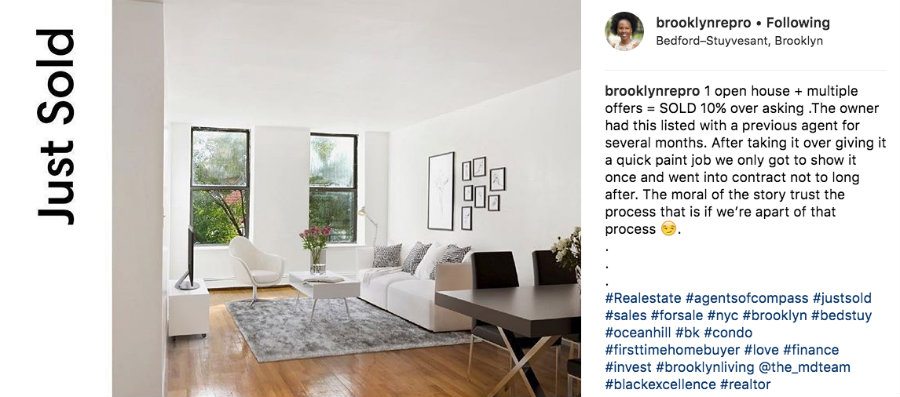A pristine interior view showcases a house with gleaming hardwood floors, exuding a sense of cleanliness and modernity. To the right of the image is the profile picture of an African American woman, likely the real estate agent responsible for the sale. The accompanying description details the impressive achievement of selling the Brooklyn property at 10% above the asking price after a single open house. The house had been listed with another agent for several months with no success. However, after a quick paint job and a single showing, the property quickly went under contract. The caption concludes with an encouraging note to "trust the process" when the agent is involved, followed by a cheerful smiley face emoji. Relevant hashtags include #RealEstate, #AgentsOfCompass, #JustSold, #Sales, #ForSale, #NYC, and #Brooklyn.